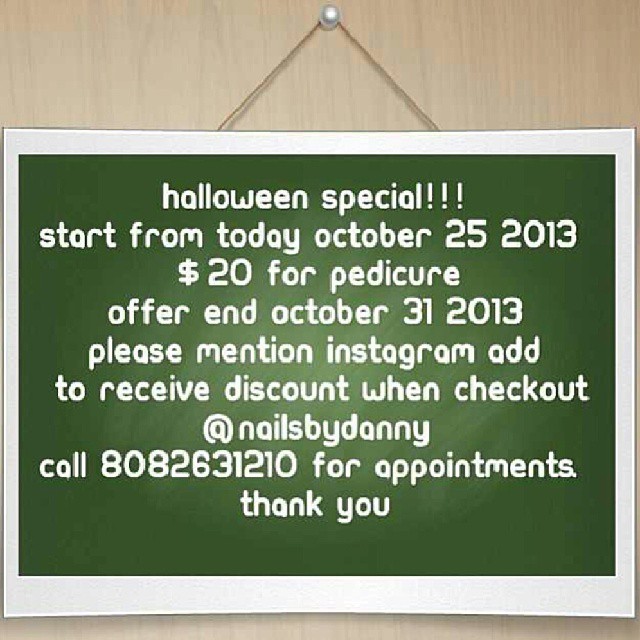The image features a digitally created graphic designed to resemble a sign hanging from a wall adorned with light beechwood paneling, displaying a prominent wood grain pattern in a tan hue. Suspended from a metallic pearl-like thumbtack, a piece of thin twine holds up a square green sign bordered in white. The sign, designed to mimic a green chalkboard, contains detailed white text promoting a special Halloween offer. The message reads: "Halloween Special! Start from today, October 25, 2013. $20 for pedicure. Offer ends October 31, 2013. Please mention Instagram ad to receive discount when checking out at Nails by Dani. Call 808-263-1210 for appointments. Thank you." Notably, the word "ad" is mistakenly spelled as "A-D-D."